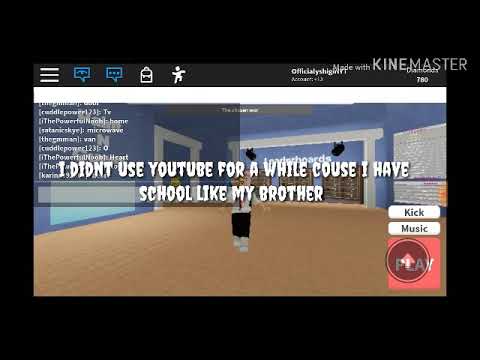The screenshot is likely from a mobile, cartoonish game featuring a small, blackish character wearing black pants, a white shirt, and white shoes. The setting is an empty room with a beige floor, blue walls, and white door frames. The upper portion of the screen displays a menu bar with icons, including a running person, indicating various menu options. Overlaid text at the center reads, "I didn't use YouTube for a while cuz I have school like my brother," with some spelling inconsistencies. In the top right corner, there is a watermark that says "KineMaster," likely the screen capture software. In the bottom right corner, there is a red button labeled "kick," alongside options for "music" and "play," suggesting in-game controls. The room features white trim along the entryways and a couple of spotlights attached to the upper trim, and the character appears to be dancing or in motion.